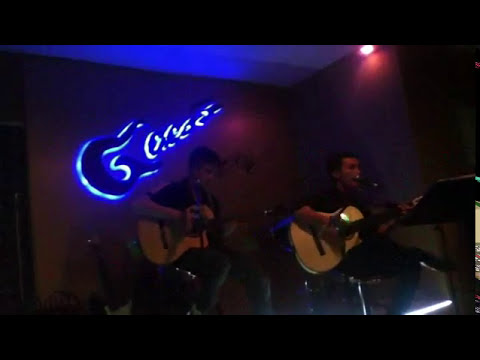In this somewhat dark and slightly unclear photograph, two young white men are seated on a stage, each holding a light beige guitar and seemingly engrossed in their performance. Both are dressed in black clothing, with the man on the left wearing black top and blue jeans and the one on the right clad entirely in black, including his shoes. They are sitting in chairs and appear to be playing right-handed guitars. Positioned centrally in the image, both performers have microphones in front of them, pointing to the likelihood that they are singing for an audience. A music stand is placed to the right of the man on the right. The backdrop is a dark red, possibly wooden wall, featuring a blue neon sign with indistinct lettering, though the first letter might be a G. There is also an additional guitar standing against the wall near them. The setting resembles a dimly lit studio or possibly a performance space within a restaurant, suggested by the ambient mix of colors like black, brown, blue, white, pink, orange, red, tan, and gray. A reddish light beam spotlights the man on the right, emphasizing the intimate and atmospheric mood of the scene.